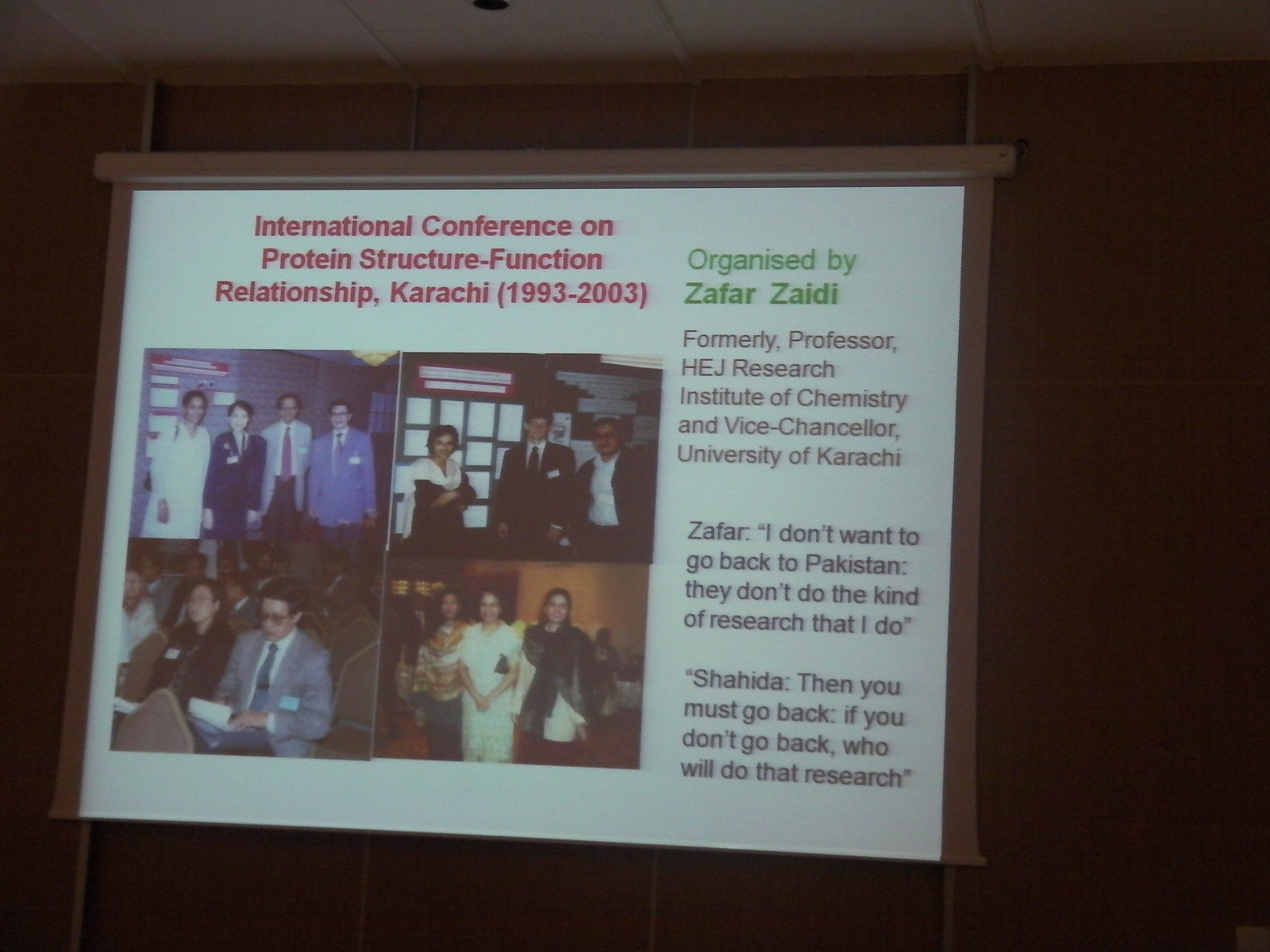The image is of a slightly out-of-focus, framed plaque or poster mounted on a paneled wooden wall, with the background showing vertical panels and a glimpse of a light-colored ceiling at the top. The poster itself has a wooden frame on the top and sides but not at the bottom. The prominent headline, printed in three lines of red text, reads: "International Conference on Protein Structure Function Relationship Karachi (1993 to 2003)." Below the headline are four photographs arranged in a grid, with two on the top row and two on the bottom. The top left photograph shows four individuals facing the camera, while the top right photograph features three people also facing forward. The bottom left photo captures a group of people seated in rows, with two individuals prominently visible. The bottom right photograph depicts three women posing for a picture. To the right of these photos, in two lines of green text, it says, "Organized by Zafar Zaidi," followed by three paragraphs of black text. Zafar Zaidi is mentioned as a former professor at the HEJ Research Institute of Chemistry and Vice Chancellor of the University of Karachi. A notable quote in the text highlights a conversation where Zafar says, "I don't want to go back to Pakistan. They don't do the kind of research that I do," to which Shahida responds, "Then you must go back. If you don't go back, who will do that research?" The participants in the photos are dressed in formal attire, including sport coats and fancy dresses, and some are seen wearing name tags suggestive of a conference or convention.